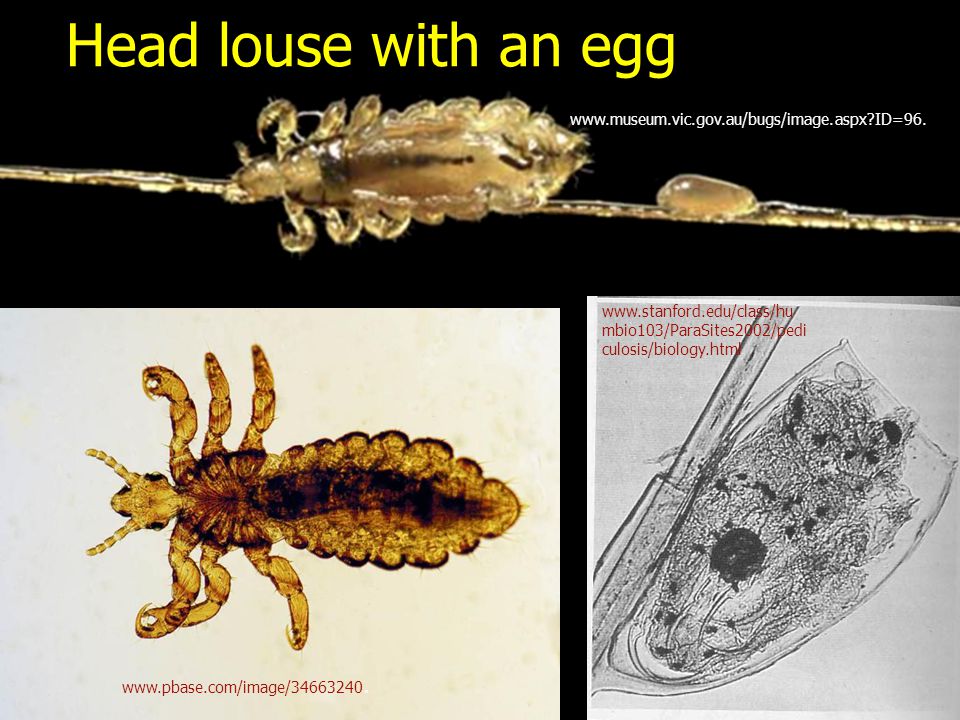A composite image features three sections depicting various views of a head louse. At the top, a clear, horizontally oriented photograph shows a head louse with an egg attached to a brown hair strand. The yellow caption above reads, "Head louse with an egg," while the accompanying website address, "www.museum.vic.gov.au/bugs/image.aspx?id=96," is prominently displayed. The louse in this image is yellowish in color, with a distinct segmented body, six legs, and two antennae, next to a droplet-like structure.

The bottom-left section portrays a top-down view of a similar louse, more darkly colored, possibly casting a darker, more saturated brown. Its three pairs of legs and antennae are clearly visible against a contrasting white background. Below this image is the website "www.pba.org.au." 

On the bottom right, a high-contrast, black-and-white microscopic image showcases another perspective of the louse. This segment's details are more abstract and intricate, likely emphasizing the biological structure of the louse. The associated URL, "www.stanford.edu/class/humbl0103/parasites2002/pediculosis/biology.html," is printed above in red against a grayish-white backdrop.